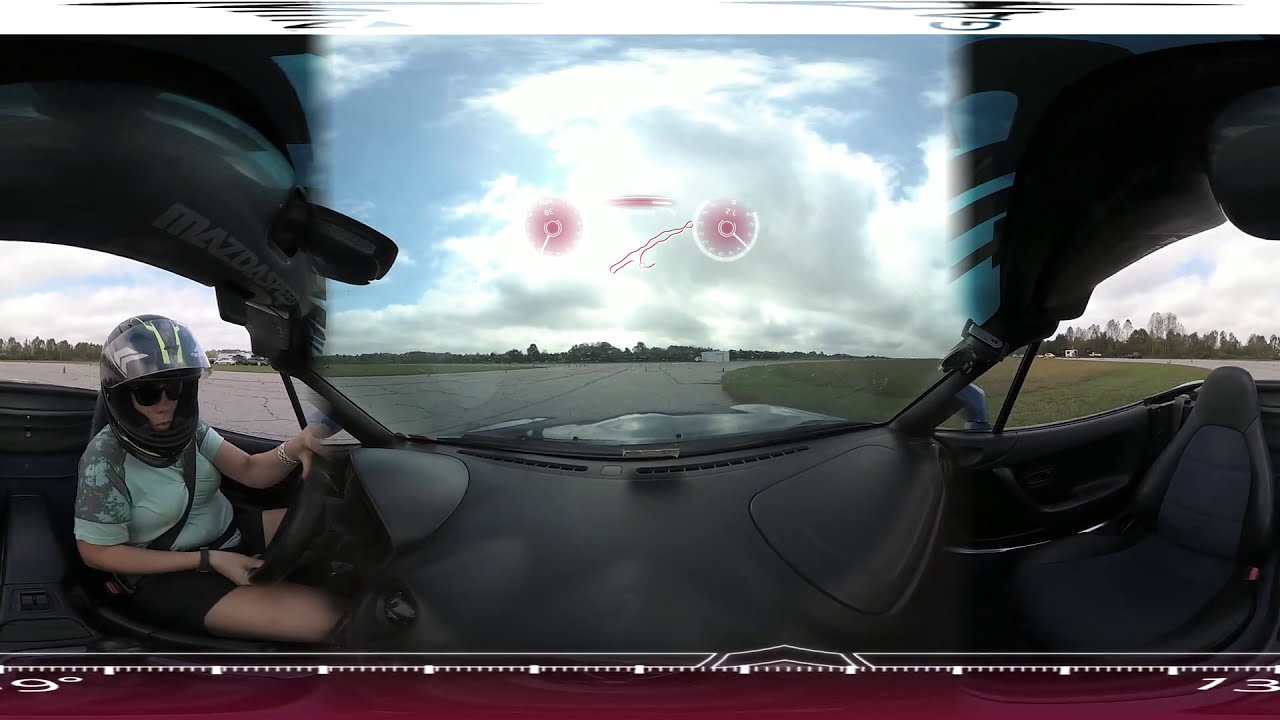In this dynamic and immersive fisheye-lens photograph taken at a racetrack, we see a woman expertly maneuvering a Mazda car. The photograph, possibly captured using a 360-degree camera, stitches together multiple perspectives, warping the image and providing a comprehensive view of both the driver and the interior of the vehicle. 

The woman, positioned on the left side of the image, is wearing a light mint green shirt adorned with a subtle floral design on the shoulders, black shorts, and a black racing helmet with the visor flipped up. Her eyes are shielded by black sunglasses, projecting confidence and focus. She grips the steering wheel with both hands, revealing a watch on her right wrist and a bracelet on her left. The car's interior is sleek and predominantly black, featuring ergonomic bucket seats that add to the intense racing atmosphere.

Above, the sun visor prominently displays “Mazda Speed,” affirming the car's make. The photograph captures the blue sky dotted with gray and white clouds, suggesting fair weather. The racetrack stretches out ahead with minor cracks visible in the pavement, surrounded by flat, green grass and a backdrop of lush trees, invoking a warm summer day. Centrally displayed digital gauges and a GPS layout of the track hover at the top of the image, heightening the sense of speed and precision driving.